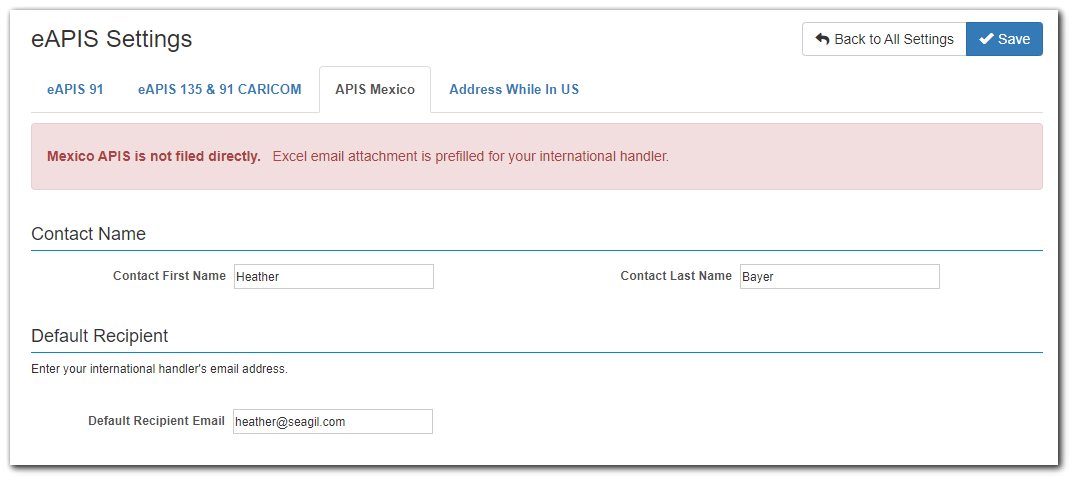In the EAPIS user interface, the settings for the system are displayed predominantly in black, with "EAPIS 91" highlighted in blue. There are various tabs to navigate through, and currently, the user is focused on the "APIS Mexico" tab. The selected "EAPIS 91" setting stands out prominently in black, whereas the others are aligned more flush with the interface.

At the top right corner, there's a "Back to All Settings" button in white, featuring a leftward-pointing arrow, labeled simply as "Back." Adjacent to it is a blue "Save" button with a check mark, designed for confirming any changes made.

Beneath these buttons, a pink box with red writing alerts users that "Mexico APIS is not filed directly." This notification is bolded and specifies that it is emailed as Excel attachments, pre-filled for international handlers.

Further down, the interface requests a "Contact Name" in a sizeable black font, followed by a blue line extending to the right. Below this line, the form requests specific details: "Contact First Name" with a text box containing "Heather," followed by "Contact Last Name" to the right, with the text box containing "Bayer."

Continuing in the same format and text size, another section labeled "Default Recipient" asks for an email address, suggesting either the user's email or that of an international handler. The "Default Recipient Email" is provided as "heather@seagold.com," displayed in a plain white text box.